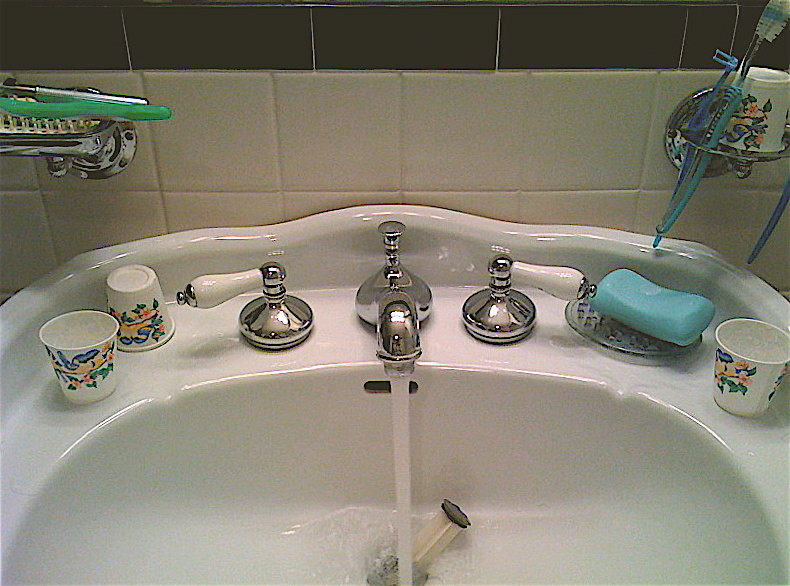The image captures a detailed view of a home bathroom. At the top of the picture, there's a row of black tiles with white grout. Beneath these, two white tiles with matching white grout are visible. Positioned on the upper left is a silver holder embedded into the tiles, potentially used for holding a toothbrush, while on the right, another holder cradles a translucent blue or green toothbrush, accompanied by a small Dixie cup.

The sink itself is white with an undulating, wavy edge pattern that creates a dynamic visual flow. Water gushes out at full blast from a silver faucet, which is complemented by white handles. On the left side of the sink, two Dixie cups with green and yellow designs are arranged—one facing up and the other down. To the right of the sink, a small rubber mat holds a piece of blue soap, adjacent to another upright Dixie cup. Intriguingly, a piece of plastic is protruding from the sink's drain, adding an unexpected element to the scene.